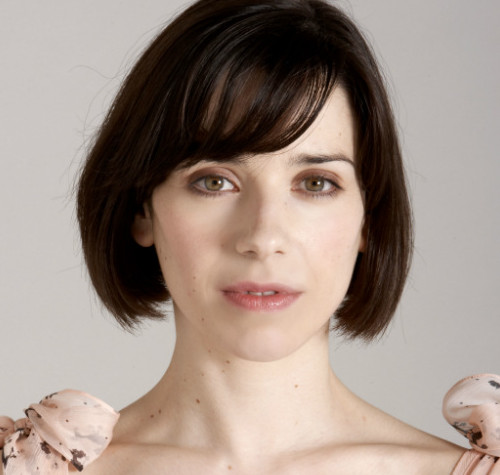In this professional, indoor studio shot, a young woman with a bob haircut and bangs is positioned directly in the center of the image against a lighted white or possibly gray background. She has straight brown hair, fair skin, and hazel eyes adorned with subtle brown eyeshadow and minimal eye makeup. Her expression appears to be one of subdued amusement without a pronounced smile. Notably, she is wearing poofy, pale pink ribbons on her shoulders, which are visible at the corners of the image. The photo, restricted to her head and neck, also shows numerous beauty marks on her neck and her piercined lips. Her hair slightly obscures her left eye while leaving her right eye completely visible. The overall aesthetic of the image is notably light and fair, dominated by white and pale shades intersected by the brown of her hair.